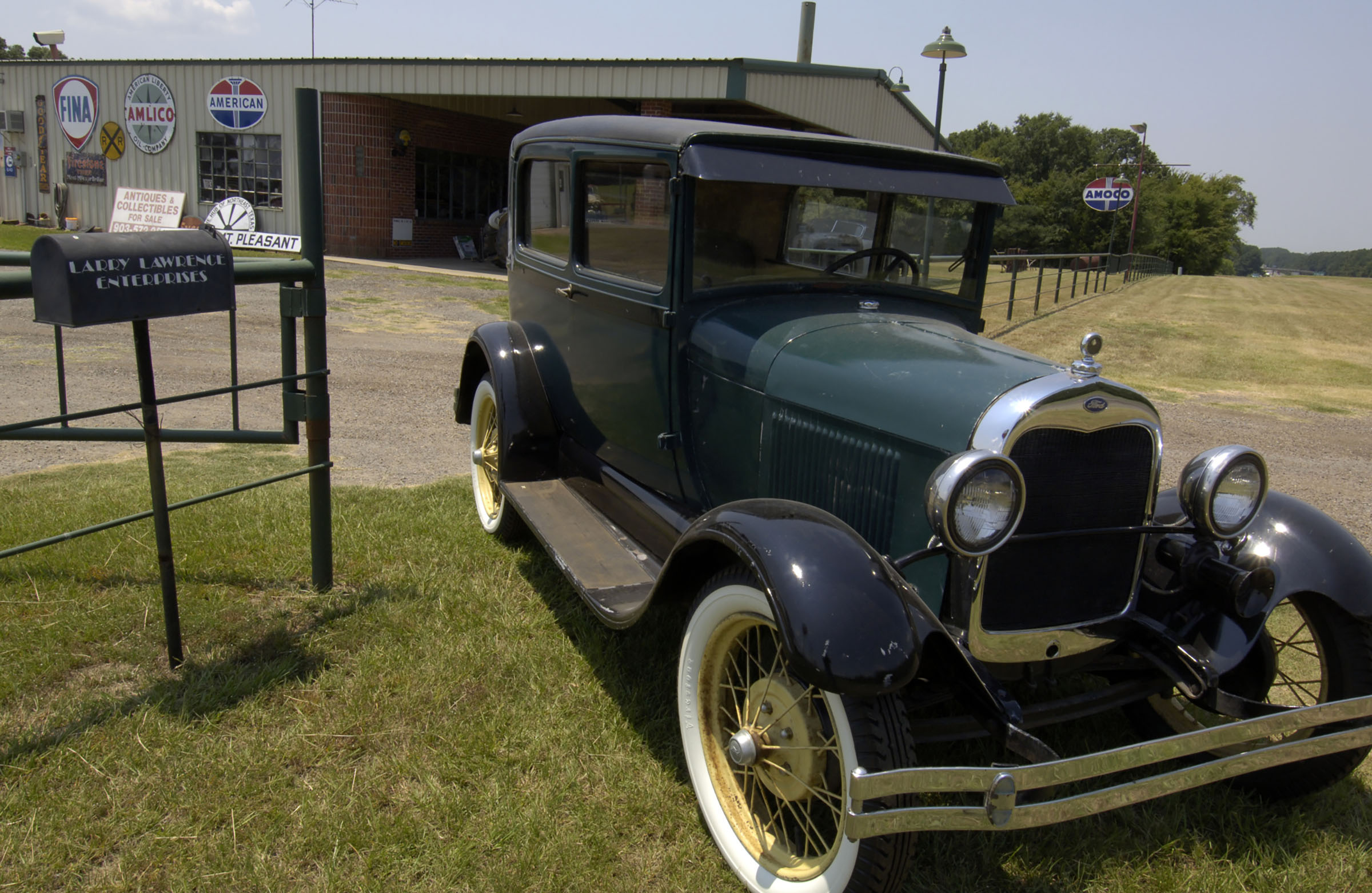The photograph captures a vibrant scene of a vintage 1930s roadster parked diagonally in the bottom right-hand corner on a patch of grass. The car, predominantly black with a square-type cab and gold-spoked wheels surrounded by white wall tires, features a long hood and a metal front bumper. A gray mailbox bearing the inscription “Larry Lawrence Enterprises” stands to the left side of the car, though one caption suggests it may read "Sally Lawrence Collection." Behind the car lies a dirt gravel driveway leading to a single-story gray building adorned with several nostalgic signs: a circular gray "Amlico" sign, a red, white, and blue “American” sign, a shield-shaped "FINA" sign, and a larger "Amoco" sign visible in the background. Complementing the setting are elements like a “Mount Pleasant” sign leaning against the building, along with scattered street lamps, a protective fence, and lush trees under a clear blue sky, suggesting a bright, sunny day. This picturesque outdoor scene wonderfully merges elements of past automotive design and classic Americana signage.